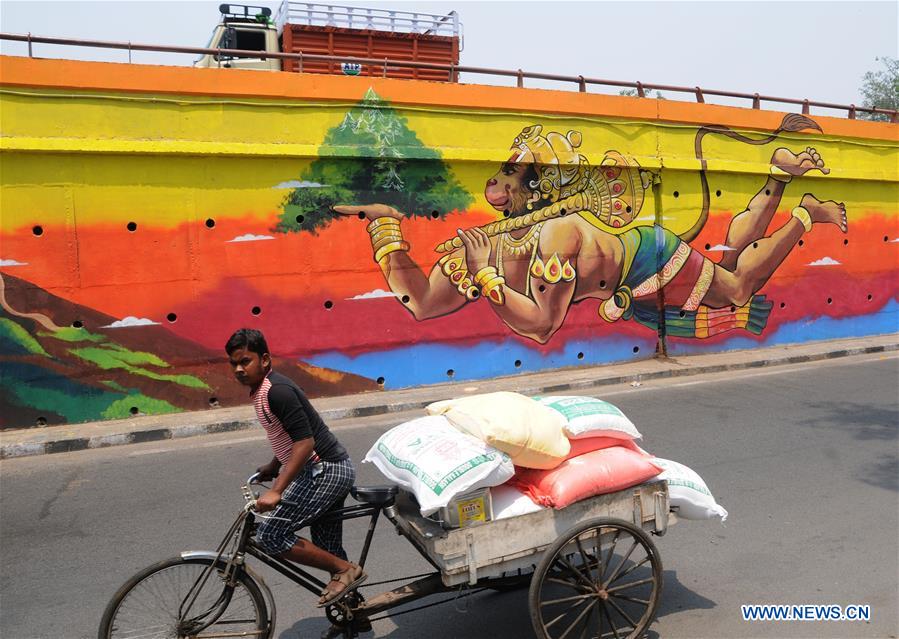In the photograph, a young man of Southeast Asian descent is captured bicycling past a detailed and colorful wall mural. He has dark hair and is wearing a three-quarter length sleeve top that is black and red, paired with plaid shorts and sandals. The man is glaring at the camera while riding a black bicycle, which has an attached cart loaded with several bags. The bags, which appear to be holding grains or similar goods, are in various colors including white, green, yellow, and red.

The mural behind him is vibrant and intricate, seemingly attached to a bridge or roadway, as there is a yellow truck with a red trailer visible above it. The mural depicts a divine figure that appears to be a god with partial monkey features, adorned in traditional Indian attire with abundant gold jewelry. The figure is holding a large golden staff and lifting a tree, while wearing a colorful sarong that features green, blue, and red hues. The mural combines elements of yellow, orange, and red, adding to its vivid and animated appearance.